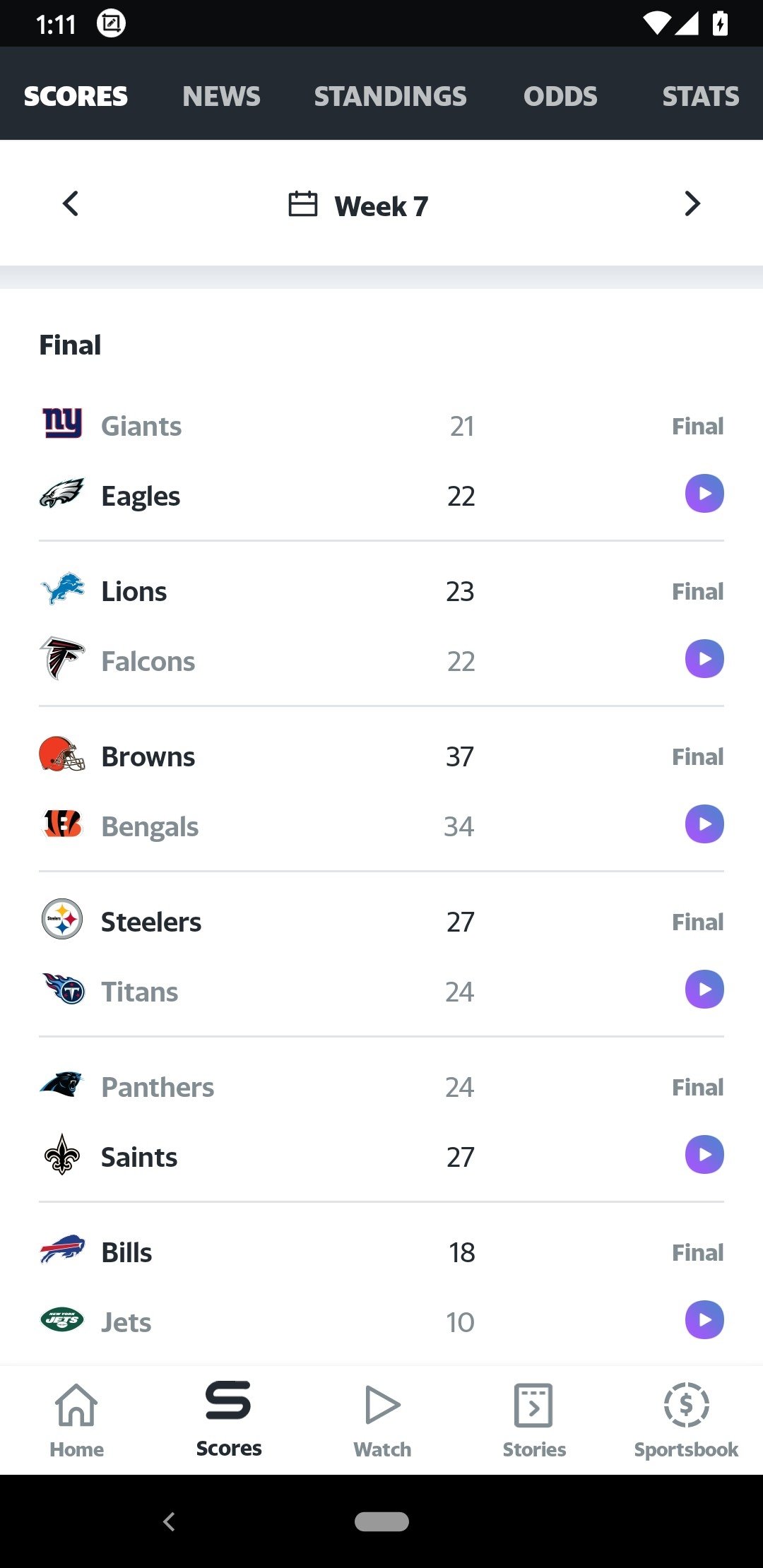The image is a screenshot showcasing multiple NFL games from Week 7, displayed on an organized scoreboard interface. At the top of the scoreboard are various categories including Scores, News, Standings, Odds, and Stats, indicating a comprehensive overview of the league’s status. 

Prominently listed along the left side are the team logos representing different NFL franchises such as the Giants, Eagles, Lions, Falcons, Browns, Bengals, Steelers, Titans, Panthers, Saints, Bills, and Jets. Each logo is neatly aligned next to its corresponding team’s name.

In the center of the scoreboard, the scores of these teams are prominently displayed, offering a clear view of each game’s outcome. On the right side of the scoreboard, it is clearly indicated that all the games have concluded, as each game is marked "Final."

The scoreboard includes six different matchups, featuring a total of 12 teams. Below the scoreboard, a horizontal menu provides additional navigational options including Home, Scores, Watch, Stories, and Sportsbook, allowing users to easily access different sections.

The entire layout is set against a clean white background, with all text in black font for optimal readability. In the bottom left corner, there is a small black key, potentially for additional functionality or navigation.

Overall, this detailed scoreboard offers a comprehensive and clear presentation of NFL Week 7 results.